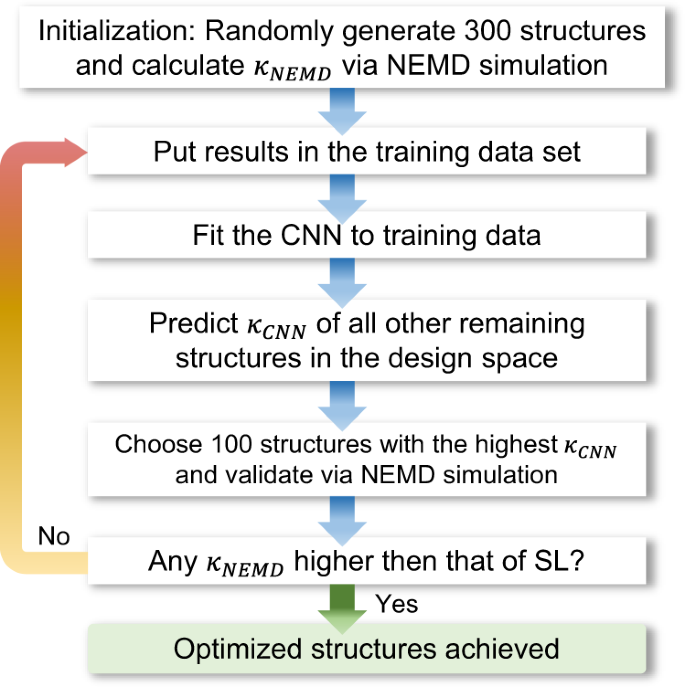This image is a detailed flowchart illustrating a multi-step procedure with distinct rectangular boxes and interconnecting arrows. Each white rectangular box contains step-by-step instructions in black text. The sequence begins at the top with the box labeled "Initialization," which instructs to "Randomly generate 300 structures and calculate KNEMD via NEMD simulation." 

A blue arrow directs to the subsequent box, "Put results in the training dataset," followed by another blue arrow leading to the box, "Fit the CNN to training data." The procedure continues with "Predict KCNN of all other remaining structures in the design space," and then moves to "Choose 100 structures with the highest KCNN and validate via NEMD simulation."

The next step questions, "Any KNEMD higher than that of SL?" Here, the path diverges: a green arrow points down to a light green box stating, "Yes, optimize structures achieved," while a yellow arrow indicates that a "No" answer loops back to the "Put results in the training dataset" step. This intricate chart ensures a clear, methodical progression for the given task.